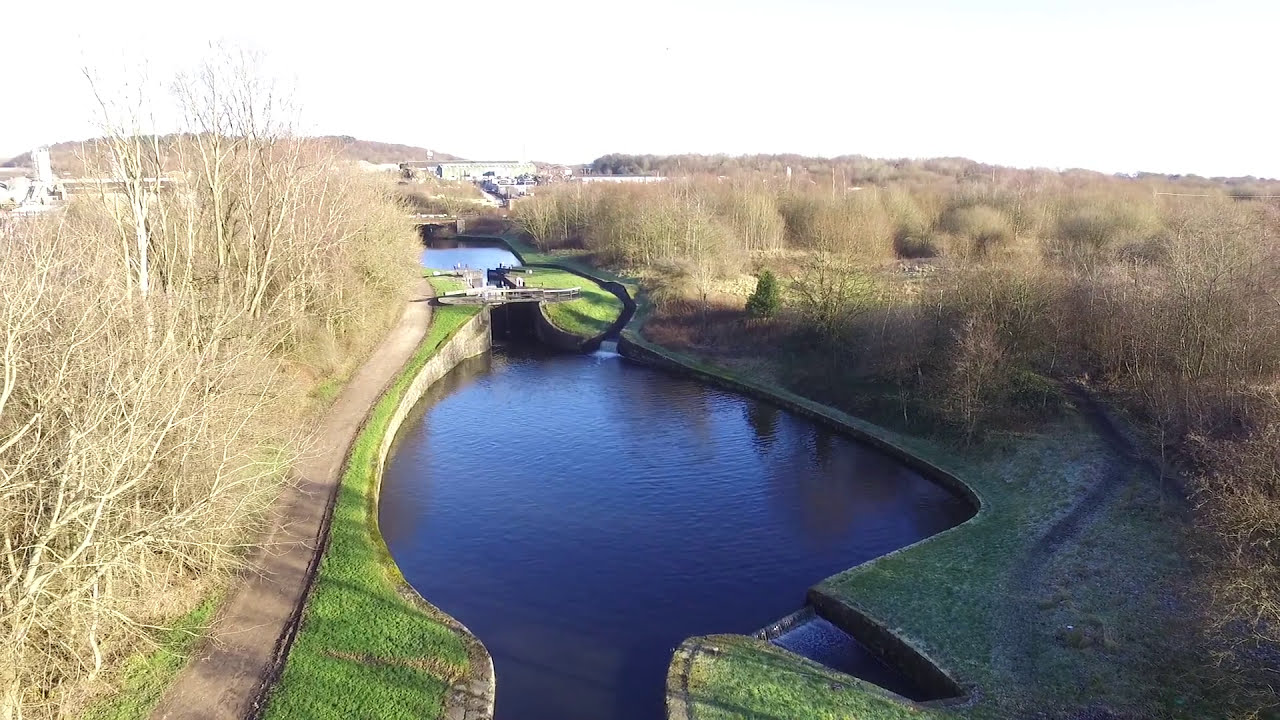The overhead shot captures an outdoor park area in late fall, evidenced by the trees on both sides of the image devoid of leaves. The sky overhead is a bright, almost white hue, casting a well-lit scene below. A prominent feature of the landscape is a man-made waterway bordered by a cement and stone structure, curving irregularly through the park, eventually opening into a pond. The water appears very still and dark blue. A bridge crosses the narrowest part near the top of this waterway, and nearby, there is a small structure resembling a dam or a tunnel. To the left of the waterway, a clearly defined bike trail and walking path stretch diagonally from the bottom left to the top left of the image. In the background, against the slightly elevated hilly terrain, the bare trees and brown bushes frame the scene, while dirt walking trails are visible on the right-hand side, completing the tranquil yet intricate landscape.